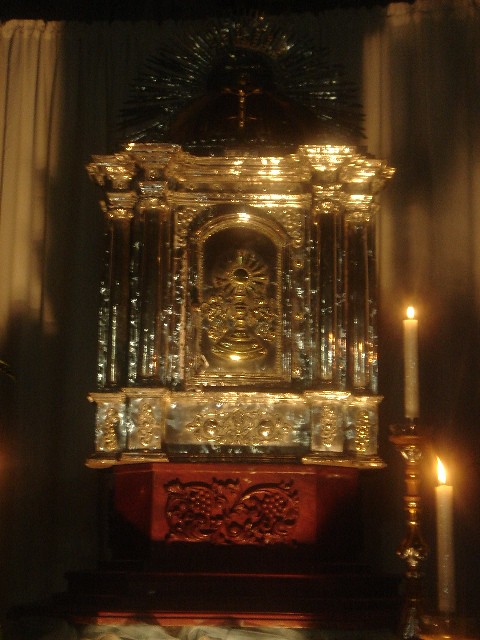The image depicts the dimly lit interior of what appears to be a church or prayer hall. Dominating the center is an ornate altar adorned with golden elements. The structure, which resembles a small palace or chapel, rests on a vibrant red platform intricately carved with images of grapes and various fruits. The golden altar features columns flanking a central emblem that includes a candlestick with a radiant ball atop it and a cross with Christ figure surrounded by thorn-like shapes at its pinnacle. Atop the altar, at the crown, there's a hint of green that may be part of a cross. The scene is bathed in the soft glow of two recently lit candles positioned to the right—one on a tall, golden candlestick, and the other on a shorter stand—casting dramatic shadows across the image. The walls in the background are shrouded in darkness, with possible curtains reflecting the candlelight, adding to the serene and solemn atmosphere.